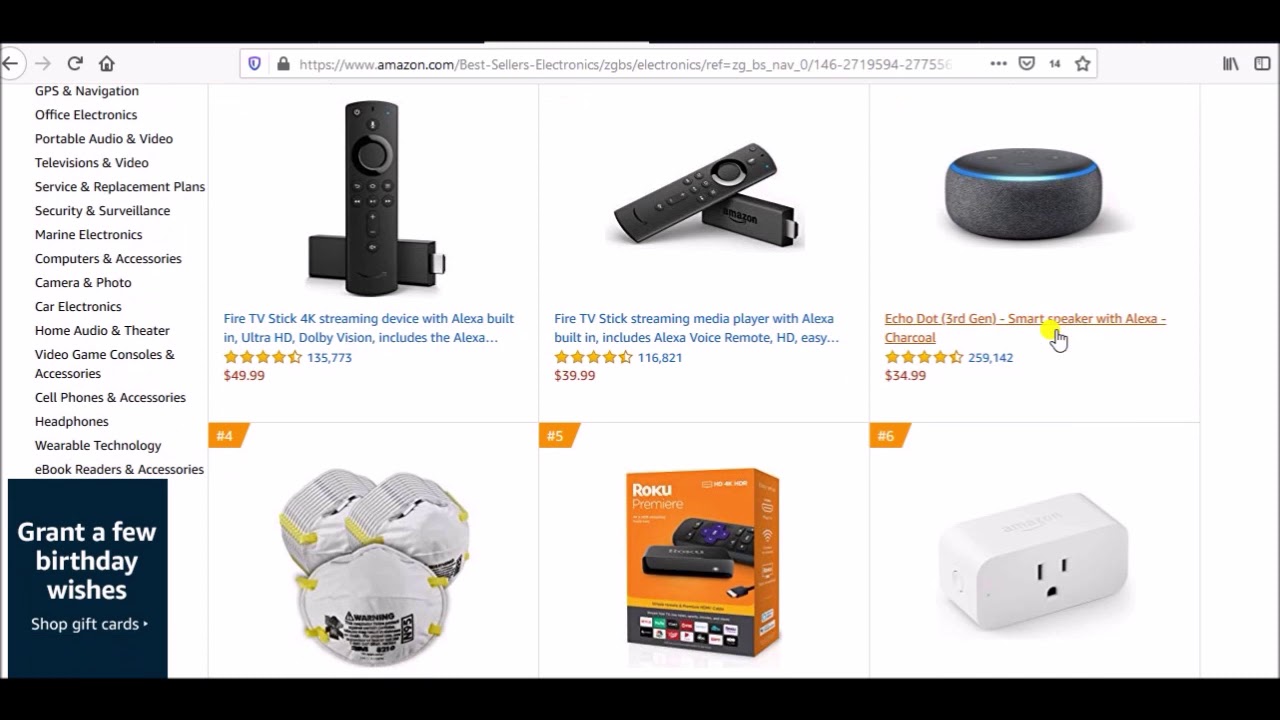This image showcases a detailed layout of Collins's product offerings and some featured electronics available for purchase. 

**Products and Categories:**
- **Far Left Section:** 
  - **Collins's GPS Navigation**
  - **Office Electronics**
  - **Portable Audio and Video**
  - **Televisions and Video**
  - **Service and Replacement Parts**
  - **Security and Surveillance**
  - **Marine Electronics**
  - **Computers and Accessories**
  - **Cameras and Photo**
  - **Car Electronics**
  - **Home Audio and Theater**
  - **Video Game Consoles and Accessories**
  - **Cell Phones and Accessories**
  - **Headphones**
  - **Wearable Technology**
  - **E-book Readers and Accessories**

In addition, there is a highlighted promotional square featuring birthday wishes and a suggestion to shop for gift cards, with a visible Amazon link to bestsellers in electronics.

**Featured Products:**
- **Fire TV:** 
  - State-of-the-art streaming media device with Alexa built-in.
  - Described as having Alexa voice control capabilities.
  - Review rating indicated as one and a half stars.

- **Fire TV Streaming Media Device:**
  - Another version highlighted with Alexa built-in.
  - It displays a four and a half gold stars rating, implying higher customer satisfaction.

- **Echo Dot (Third Generation):**
  - Smart speaker equipped with Alexa.
  - Priced at $34.99.

Additionally, there's an image of a mask and a prominent orange box featuring the Roku Premiere streaming device, with a black remote control. The Roku box suggests multiple applications available, including what appears to be an Amazon plug, all against a white background.

This comprehensive display represents an extensive range of electronics, special offers, and the latest in smart home technology.